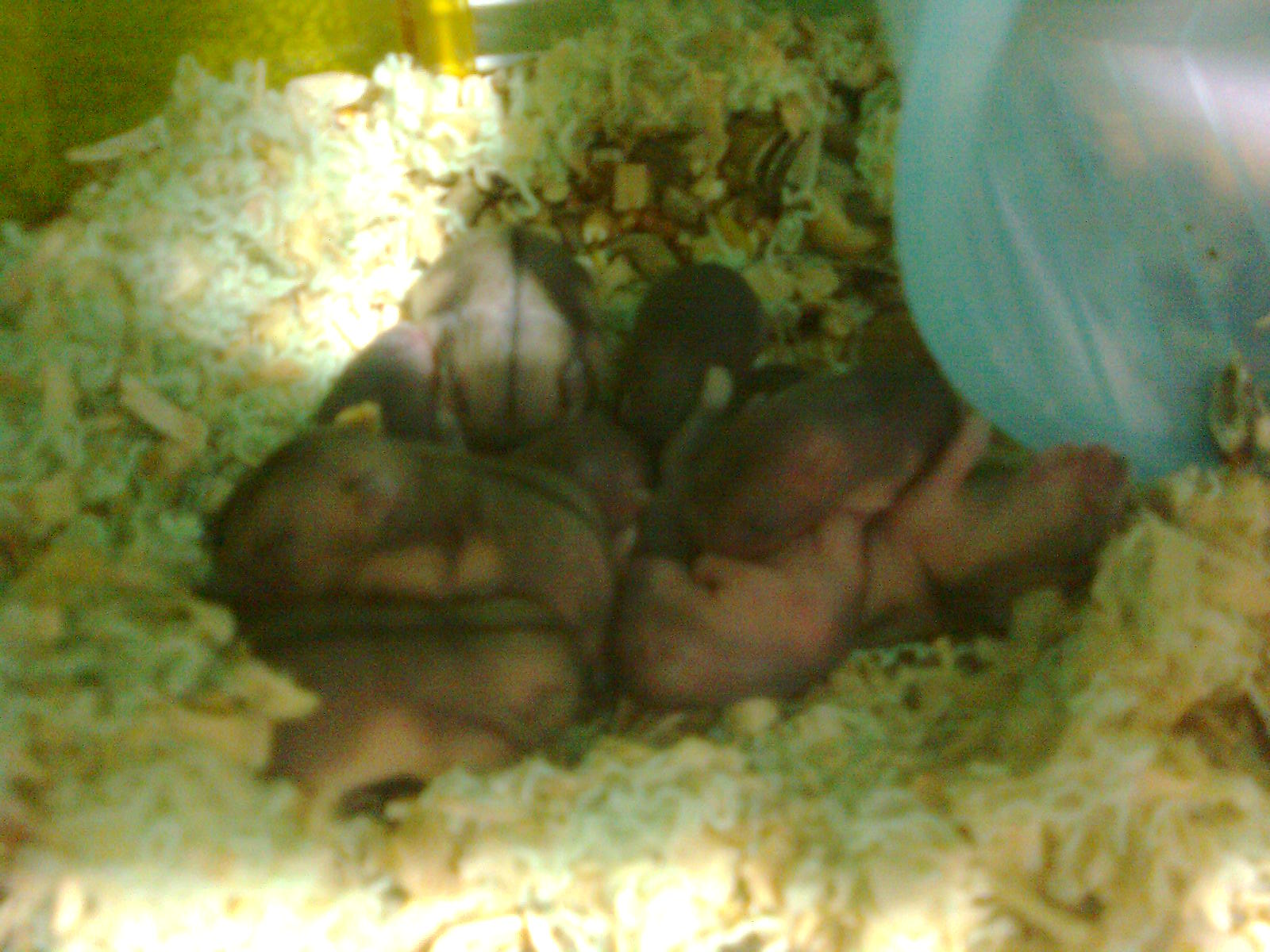The blurred color photograph appears to show a nest filled with numerous small baby animals, likely rodents such as baby hamsters or mice. The animals are dark pink with light brown shades, and many have short, sparse hair with small ears. They are lying in a nest made of wood shavings that are white and fluffy, appearing as a soft bedding. The nest itself is surrounded by some yellowish and greenish shredded materials. Within the blurred image, there seems to be a blue, translucent, rounded object, possibly a plastic tunnel or water dispenser, towards the upper right. The animals, some lying on their backs and others on their stomachs or sides, seem to be nestled together, creating a warm and secure pile. The image also contains some reflective yellow in the background, possibly suggesting elements of a cage. The overall focus of the image is poor, adding to the difficulty in identifying the exact features of the animals and objects clearly.